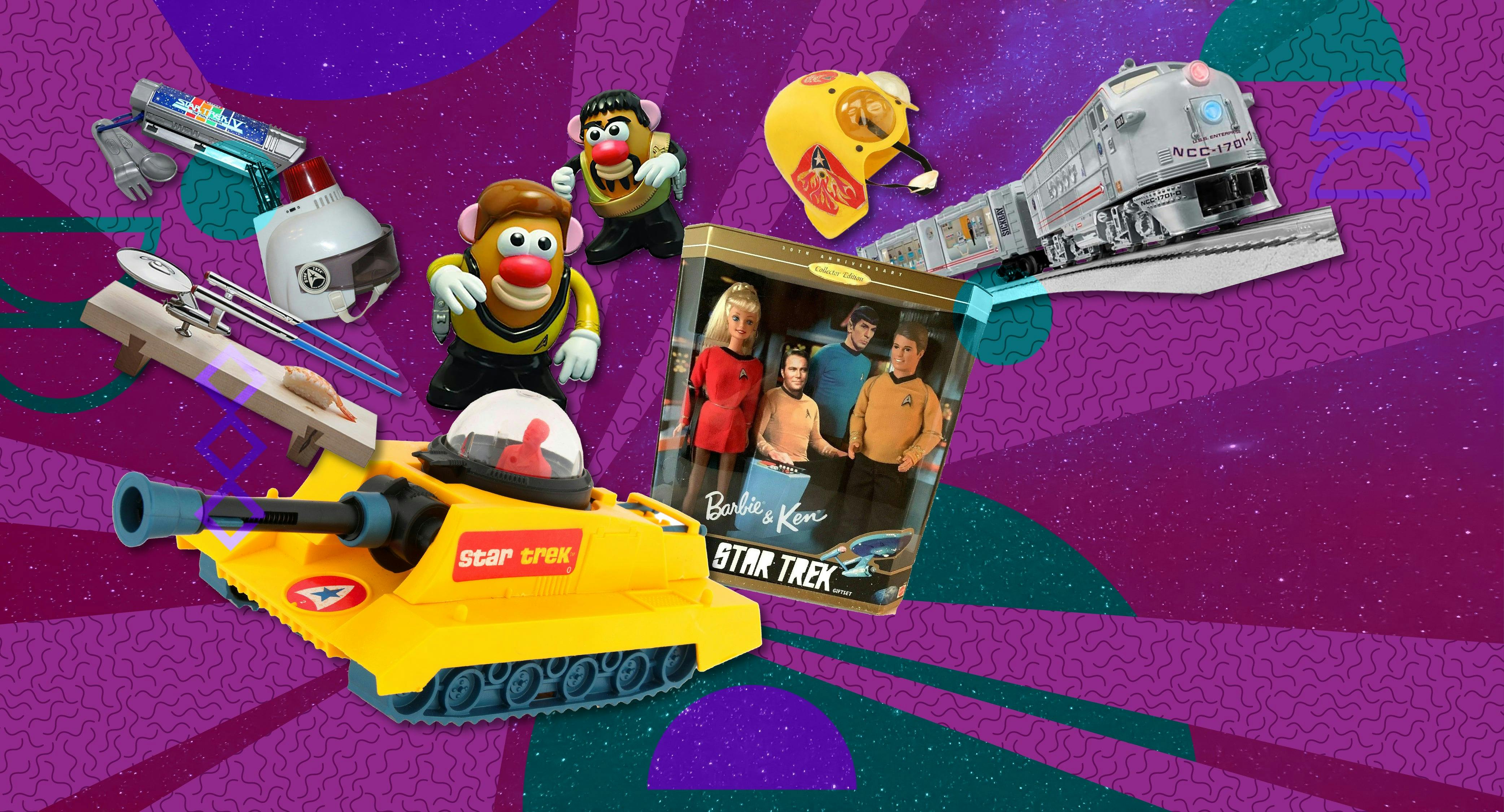This vibrant, computer-generated image features a wide horizontal rectangle with a dynamic outer space-inspired background in various shades of purple, radiating from a focal point just below center to the left. The purple hues create an effect reminiscent of the sun's rays. Interspersed within this background are additional colors like dark green, adding depth and contrast. Circular shapes, half circles, and squiggles enhance the cosmic feel.

Overlaid on this striking backdrop are an assortment of Star Trek-themed toys. A prominent yellow tank with a small figurine inside sits towards the bottom left. There is a Barbie and Ken Star Trek set, along with action figures resembling Mr. Potato Head in Star Trek attire. Spaceships, including the iconic gray USS Enterprise, and a train labeled NCC-1701D, are also featured. Additional gray plastic toys populate the scene, although their precise details are less clear. The entire composition suggests an elaborate advertisement or promotional poster, possibly for a toy store or a magazine splash page, showcasing a nostalgic collection of Star Trek memorabilia.